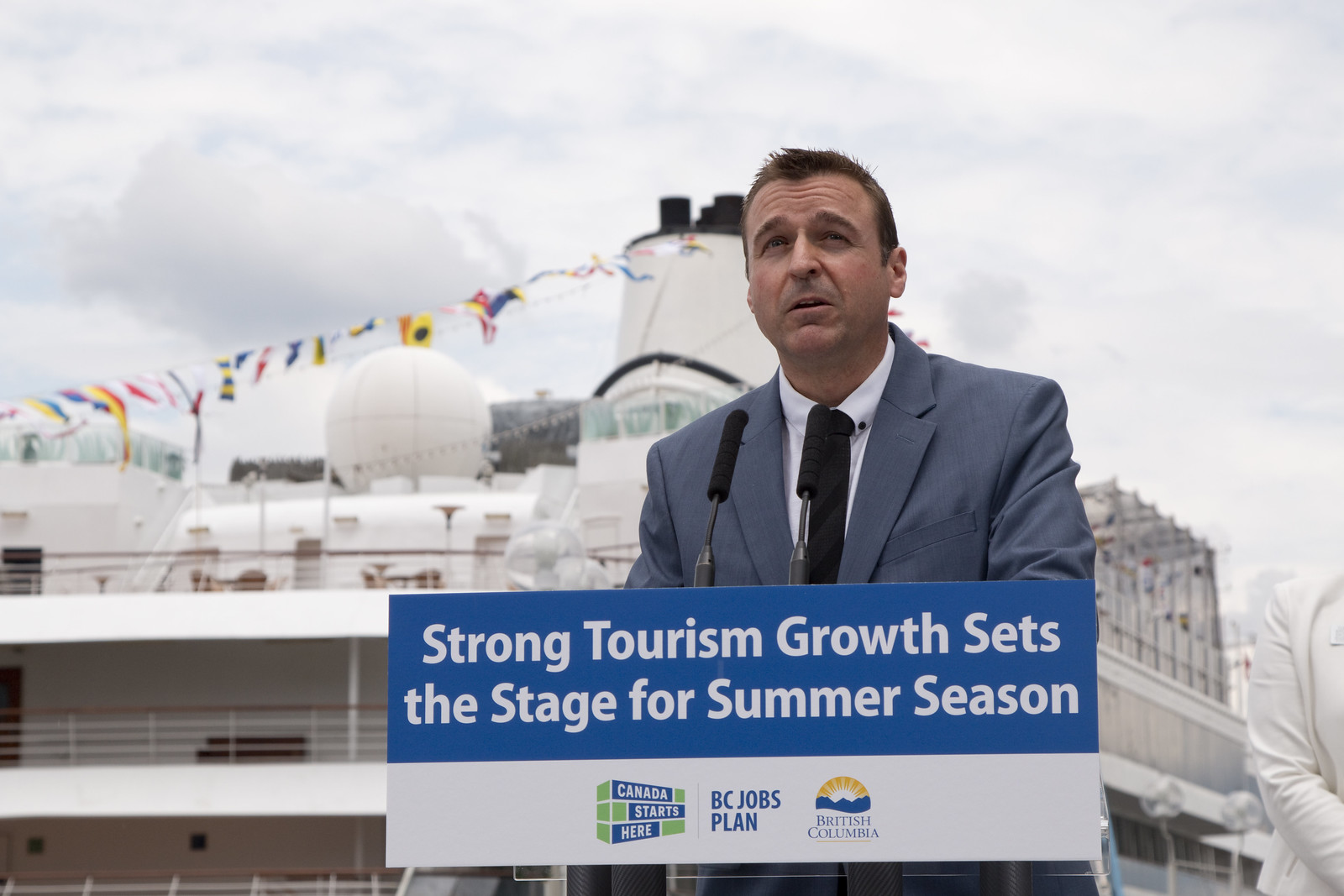This outdoor photograph captures a man delivering a speech behind a podium, set against the backdrop of what appears to be a large, multi-deck white and cream-colored building or possibly a cruise ship. The building features various white structures, smokestacks, and multicolored banners. The man, wearing a light blue suit jacket, a white shirt, and a black tie, has short light brown hair and a serious expression as he looks straight ahead. He stands behind a podium equipped with two thin black microphones. Attached to the front of the podium is a large sign that reads, "Strong tourism growth sets the stage for summer season," followed by several logos and phrases including "Canada starts here," "BC jobs plan," and "British Columbia" with its emblem. To the right of the man, a partial view of another person in white clothing is visible, though their face is not shown. The sky above is filled with clouds, adding to the dynamic atmosphere of the scene.